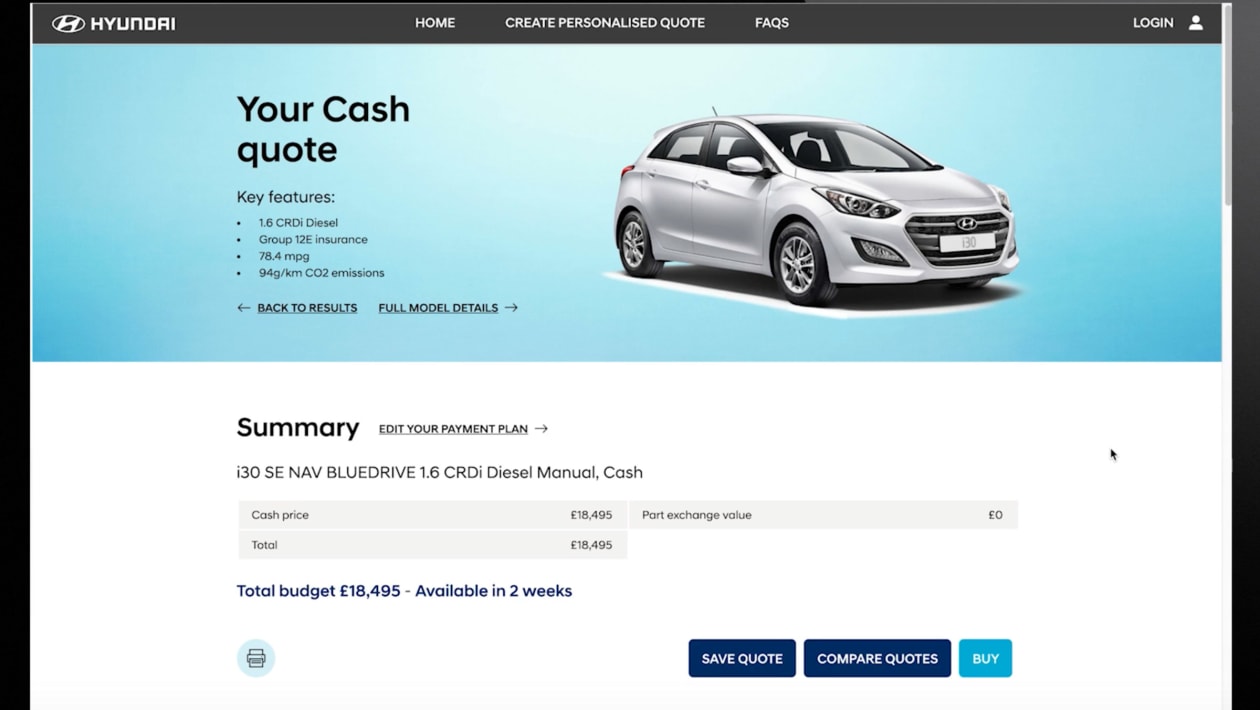The image is a horizontally rectangular screenshot of a website. At the top, there's a narrow black horizontal banner. On the left side of the banner is the Hyundai logo. Centrally located are three navigation options: "Home," "Create Personalized Quote," and "Faq." On the far right, there is a "Login" link next to a person icon that provides access to user profiles.

Below this banner, the background is light blue. On the left side, the section titled "Your Cash Quote" stands out, listing key features of the vehicle, including "1.6 CRDI diesel," "Group 12E insurance," "78.4 miles per gallon," and "94 grams per kilogram CO2 emissions."

Adjacent to this on the right side is an image of the Hyundai vehicle, which appears to be a hatchback model. Beneath the vehicle image is a section with a white background titled "Summary," accompanied by an "Edit Your Payment Plan" link. This section details the car model as "I-30 SE, NAV, Blue Drive, 1.6 CRDI, Diesel, Manual, Cash," and includes the pricing information such as "Cash Price," "Port Exchange Value," and "Total." It states that the "Total Budget" is £18,495 and mentions that the car is "available in two weeks."

At the bottom right of the image are three essential buttons: "Save Quote," "Compare Quotes," and "Buy."